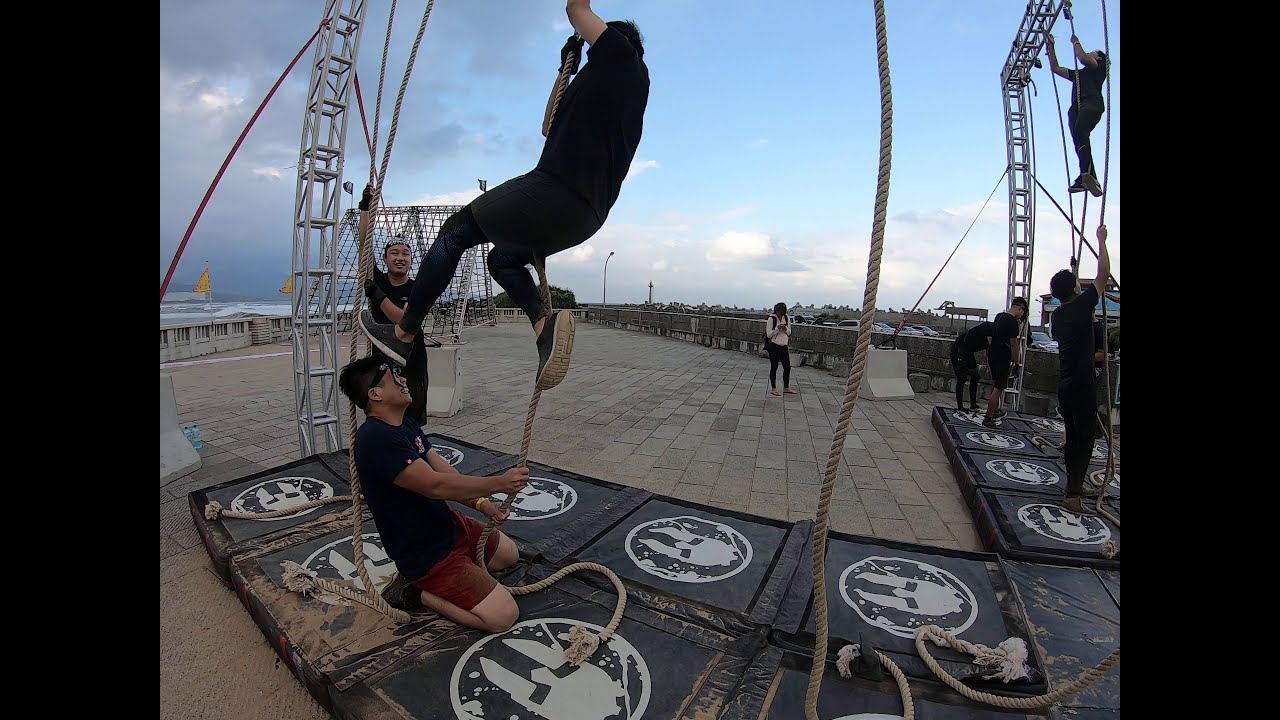In an outdoor setting by the ocean and beach visible in the top left corner, various people are engaging in a rigorous ropes course under a light blue sky with scattered white and gray clouds. They are climbing thick brown ropes that dangle from an intricate network of silver metal frames. The climbers, all uniformly dressed in black T-shirts, black shoes, and a few in black sweatpants while one man wears red shorts, navigate the ropes with one leg wrapped around and the other kicking for leverage. On the ground, large black mats with a white Spartan helmet logo centered in a circle provide cushioning below the climbers. Some individuals, including one with a white backward cap, assist by holding the ropes taut. The ground consists of grey bricks extending into the distance, while numerous climbers ascend or stabilize ropes, embodying a collective spirit reminiscent of a CrossFit team challenge.